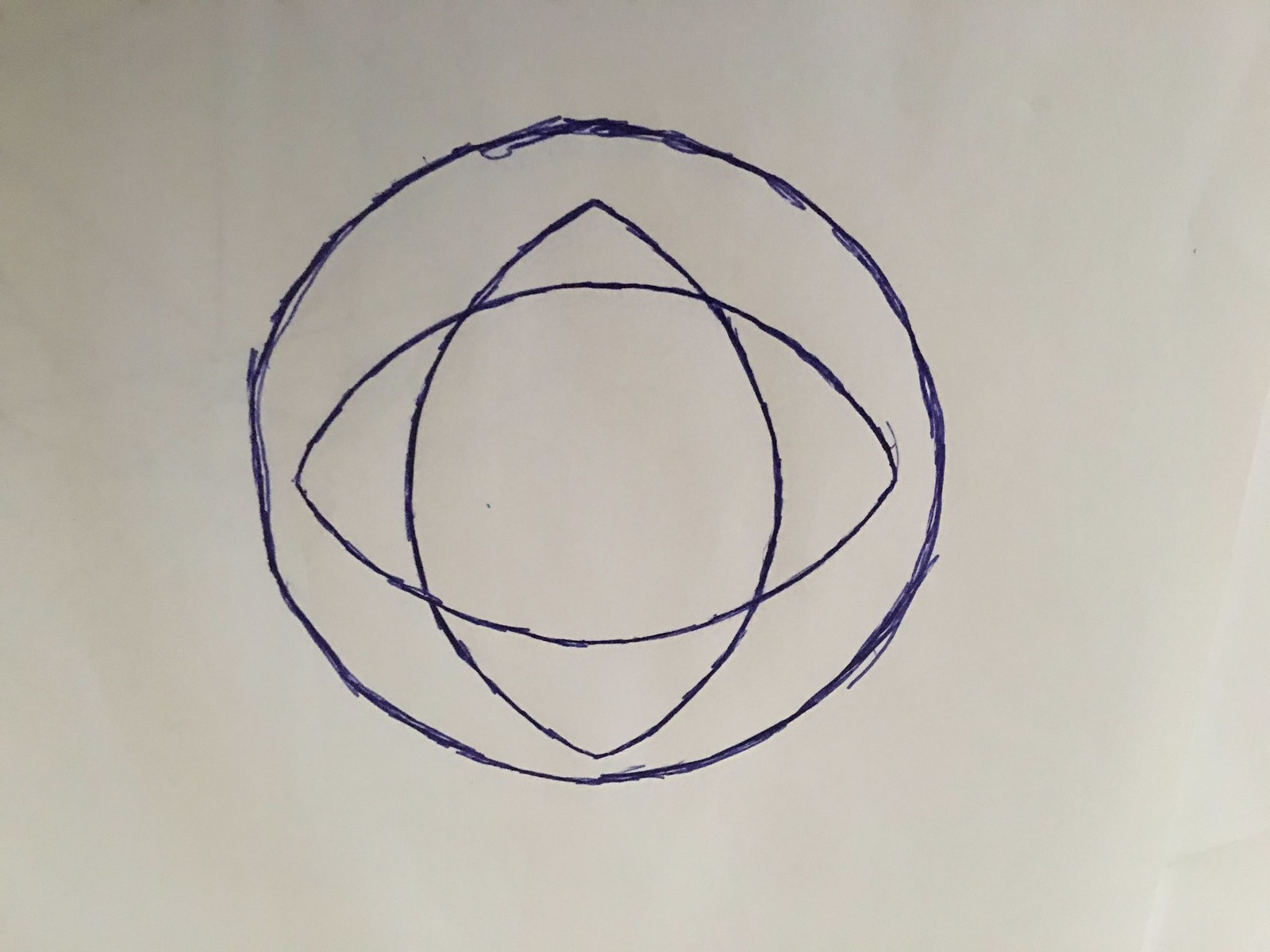This image features a blank white sheet of drawing paper that fills the entire background. In the center of the paper, slightly off to the left, there is a hand-drawn image predominantly characterized by a hollow circle. The circle, which occupies roughly 40% of the central area of the paper, has a dark blue or black outline, likely created using a pen with very dark ink. The circular outline appears imperfect and almost sketch-like, as though the artist traced over it multiple times without maintaining perfect alignment.

Inside the circle's borders, there are additional shapes, specifically two intersecting, hollow football-like forms. One shape is oriented vertically, resembling a cone standing upright, while the other is positioned horizontally, crossing the vertical shape. Both of these inner shapes are outlined in the same dark blue color as the circle and remain uncolored within their outlines. The overall composition gives a rough, organic feel as if the artist was experimenting with repeated lines and intersecting forms.